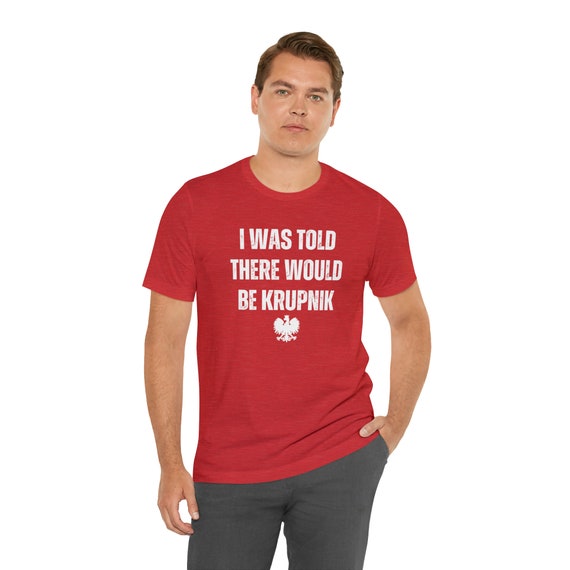A man in his 30s, with fair skin and short light brown hair, is confidently modeling against a completely white background. He stands posed and looking directly at the camera, exuding a cool and composed demeanor typical of a professional model. Clad in a snug-fitting red t-shirt and grey slacks, his outfit is sharply accentuated by his stance. His left hand is casually tucked into his pants pocket, with the thumb visible, while his right hand hangs loosely by his side. The red t-shirt, emblazoned in white capital letters, boldly declares, "I WAS TOLD THERE WOULD BE KRUPNIK," just above a small emblematic bird reminiscent of a crest. The image captures his full figure up to just above his knees, with no shadows disrupting the pristine white backdrop.